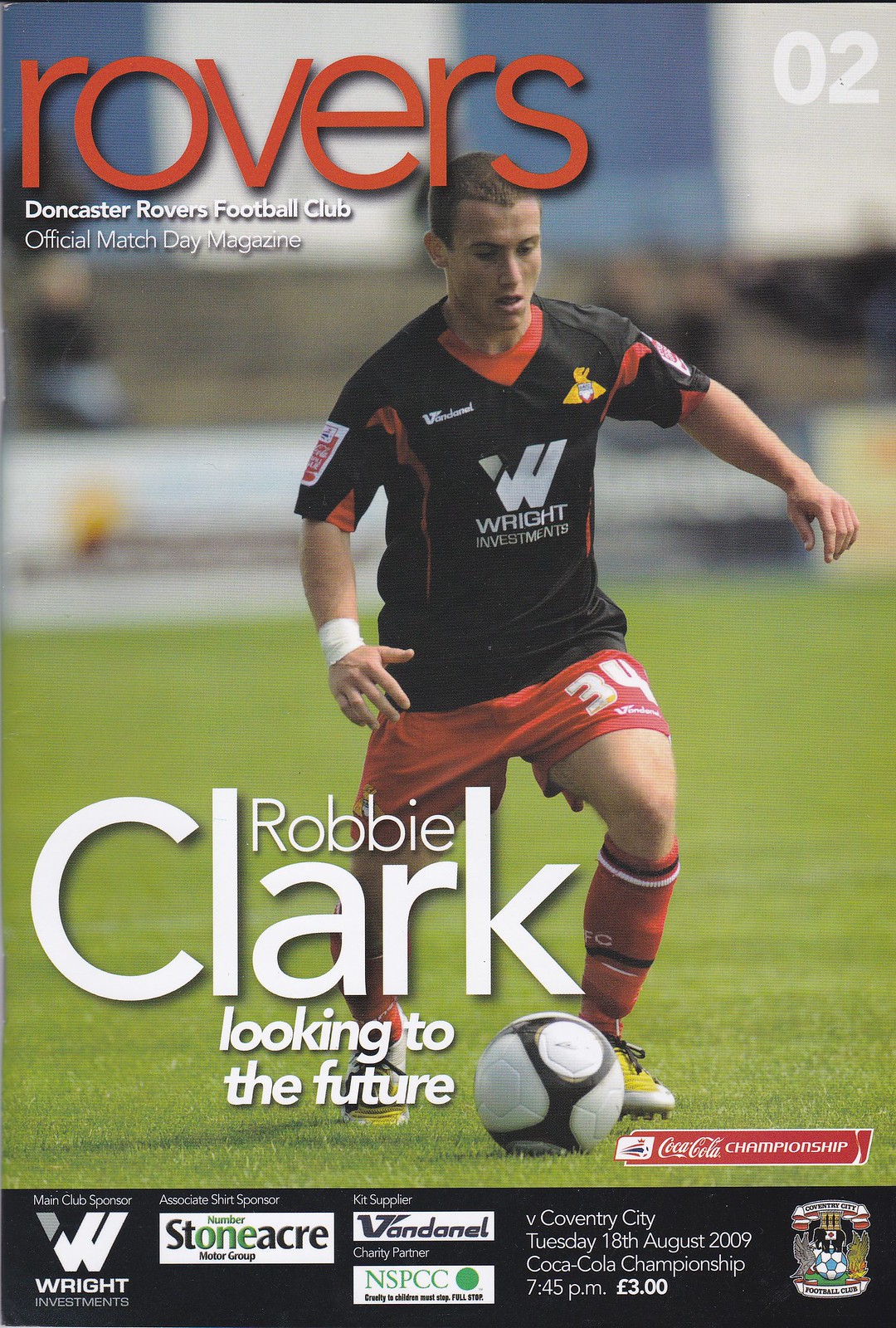The magazine cover is a vertically aligned, rectangular promotional piece showcasing a full-color photograph. It prominently features a football player named Robbie Clark. He is captured in the midst of a dynamic action shot, poised to kick a black and white soccer ball, dressed in distinctive athletic gear—red shorts emblazoned with the number 34 and a black jersey with the word "Wright" (W-R-I-G-H-T).

In the upper left corner, the word "Rovers" appears in large, lowercase red letters, beneath which "Doncaster Rovers Football Club" and "Official Match Day Magazine" are inscribed in smaller white text. The top right corner features the bold numbers "02". Below the player's image, Robbie Clark's name is highlighted; "Clark" is in large letters with "Robbie" written above the 'A' and 'R' in "Clark". A white banner near the bottom of the cover reads, "Looking to the Future," which is the title of the featured article about him.

The lower portion of the cover includes logistical details: the magazine pertains to a match against Coventry City on Tuesday, the 18th of August, 2009, part of the Coca-Cola Championship, scheduled for 7:45 PM, priced at £3. Additionally, the cover displays a banner listing the sponsors: Wright Investments, Stoneacre Market Group, Vandenelle, and NSPCC.